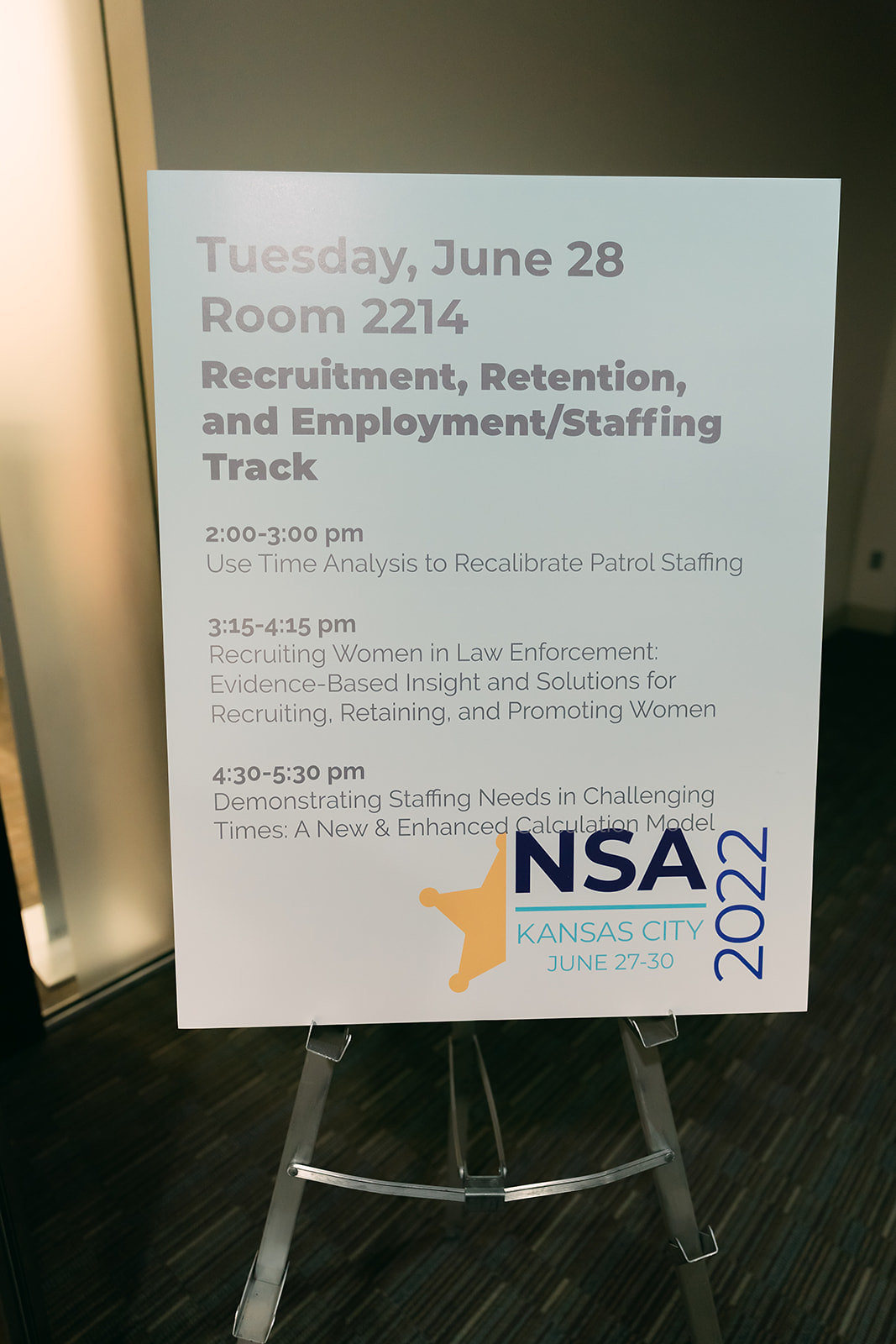The image features a large blue sign mounted on a metal tripod stand, prominently displaying information about conference sessions. The sign reads, in bold black letters, "Tuesday, June 28th, Room 2214, Recruitment, Retention, and Employment Staffing Track." It lists three sessions: "2:00 to 3:00 p.m. Use Time Analysis to Recalibrate Patrol Staffing," "3:15 to 4:15 p.m. Recruiting Women in Law Enforcement: Evidence-Based Insight and Solutions for Recruiting, Retaining, and Promoting Women," and "4:30 to 5:30 p.m. Demonstrating Staffing Needs in Challenging Times: A New Enhanced Calculation Model." Towards the bottom, it features a half-visible gold sheriff's badge, and underneath it, "NSA" in bold black print followed by "Kansas City, June 27th-30th, 2022" in purple and turquoise text. The setting appears to be a hotel conference room, indicated by the typical carpet flooring seen in such venues.